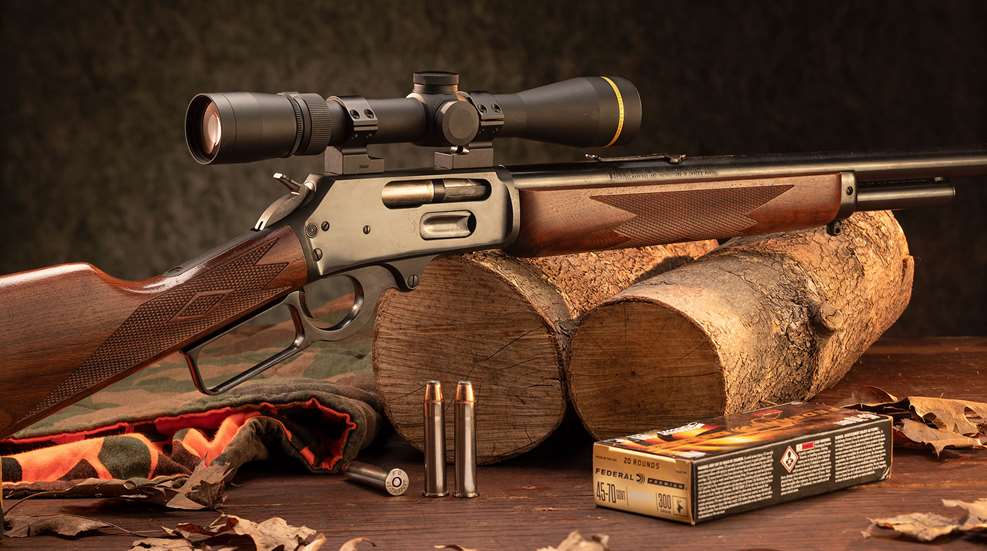This image depicts a detailed scene of a rifle setup against a stark black background. The rifle, which features a brown stock and a dark metal barrel, is elevated and stabilized by resting on two pieces of cut firewood placed on a brown wooden table. It's partially visible due to the back and front being cut off by the frame's edges. Adorning the rifle is a sizable black scope affixed on top, positioned towards the right. In the foreground, three bullets are prominently displayed – two standing upright and one lying flat. Accompanying the ammunition is a box labeled "Federal," with legible markings indicating "45-70" caliber and suggesting a quantity of 300 rounds. Scattered across the table are strips of bark or leaves, contributing to the rustic presentation, while to the side of the setup, a small rug is partially visible.